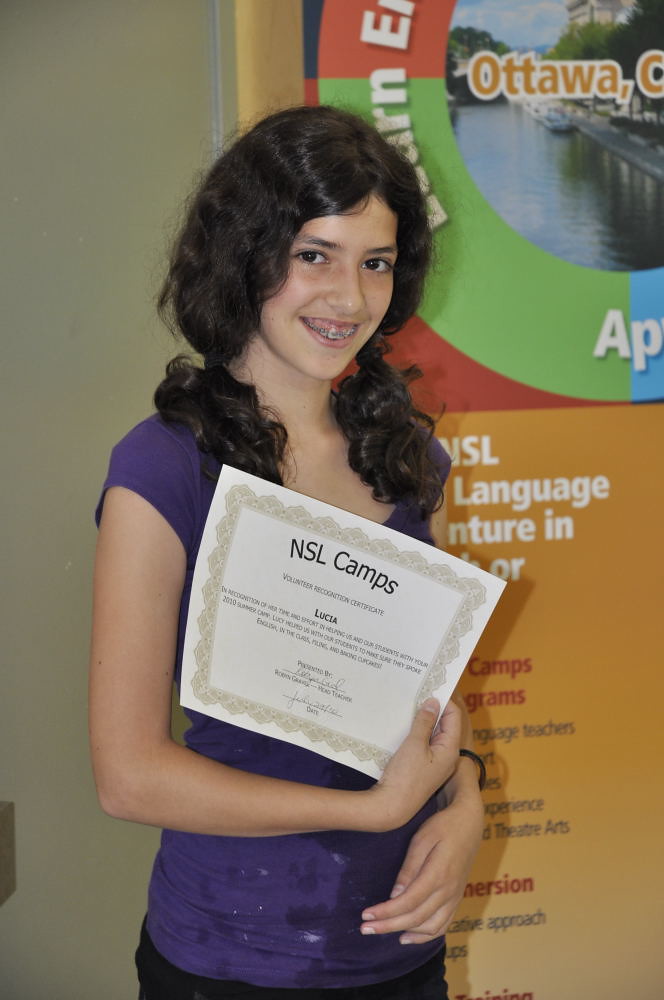This image features a young girl, likely a teenager, who appears to have a mixed heritage, possibly white and Spanish. She has nearly black, wavy hair styled into low pigtails that fall below her ears. The girl is wearing a purple t-shirt and possibly black pants, though the image ends just below her waist, making it difficult to confirm.

She is holding a certificate or award in her hands that prominently displays "NSLCAMPS" and the name "Lucia." Other text and a signature are visible but too small to read clearly. The girl has dark-colored eyes and is smiling, revealing braces on her teeth. She also wears a bracelet on her wrist.

The background includes a khaki green wall to the left and a poster on the right with an incomplete text that starts with "Ottawa." The poster features a circular, multicolored design ranging from orange to green to blue, with some letters obscured by her head. The backdrop also consists of a detailed map of Ottawa showing water, a sidewalk, and boats docked nearby, suggesting the picture might be taken in Canada. Further text on the poster includes fragmented phrases like "NSL language," "inter in camps," and "gram engaging teachers," partly obscured by her hand and the image boundaries.